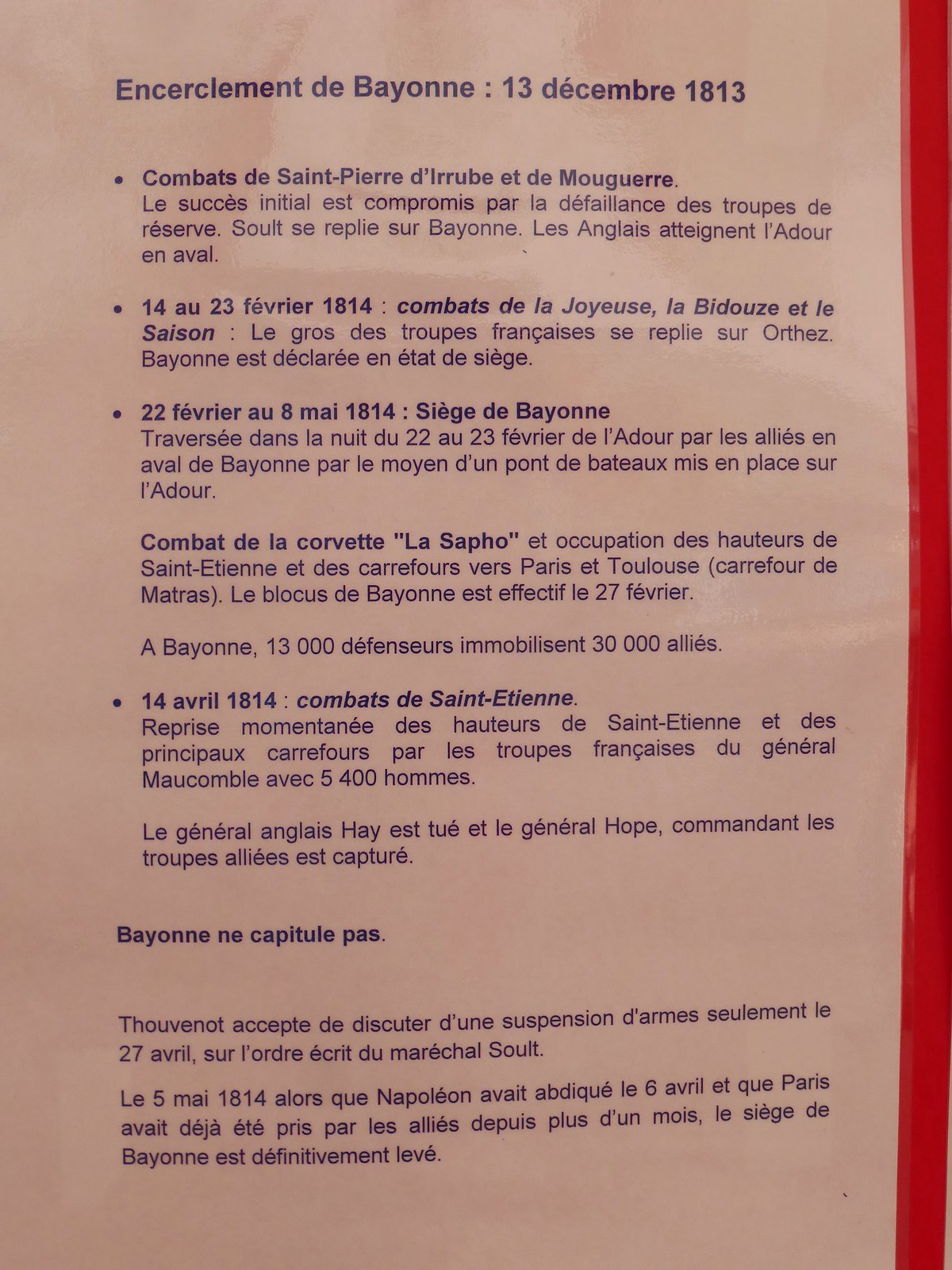The image features a white piece of paper that appears to be either taped onto a red background or laminated and then taped, exhibiting some reflections. The text on the paper is entirely in French and written in blue ink. At the very top, there is a title, "Encirclement de Bayonne, 13 December 1813," followed by four bullet points. The first bullet point reads, "Combat de Saint-Pere, Pierre de Hervé et de Muguer," and the subsequent bullet points list different dates. Below these bullet points, there is a clear separation, after which another title appears, "Bayonne Capitole Pas." Under this second title, two paragraphs of descriptive French text follow, likely summarizing the events mentioned in the bullet points.